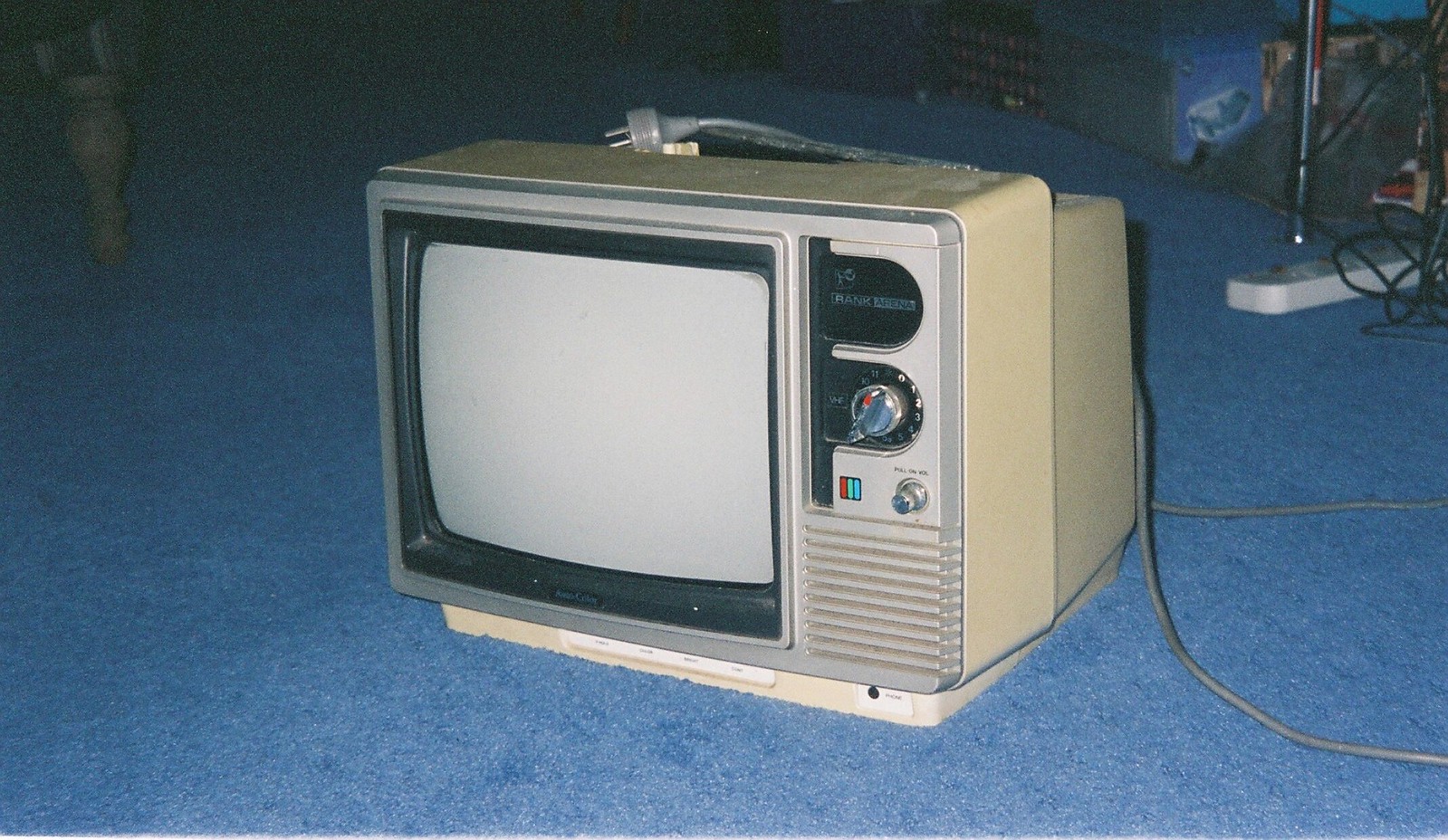The image depicts an old-fashioned Rank Arena analog television set, prominently positioned in the center. The TV, which appears to date back to the 1960s or 1970s, features a grey front with a black outline and a beige back. It is characterized by a small, blank screen, a pull-on volume switch, and a channel dial located on the right side. The top right corner of the TV displays the brand name "Rank Arena." This unplugged, boxy television is placed on a pristine, new-looking blue carpet in what appears to be a residential setting, indicated by visible furniture legs and various cables, including an electric cable extender, in the background.